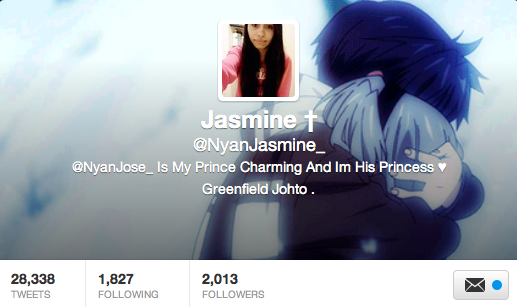The image depicts a rectangular area featuring a cloud-like background blending blue and white hues, reminiscent of an anime or cartoon style. On the right side, there are two manga characters; a boy with short brown hair is holding a girl with light blue hair, his hand placed gently on the back of her head. Overlaying this scene, in the upper to middle section, is a color photograph of a teenage girl with long black hair, wearing a pink hoodie. Below her image is text in white letters stating "Jasmine," followed by a cross, and then "@NyanJasmine." Further text reads, "@Nyan Jose is my Prince Charming and I’m his Princess Heart, Greenfield Johto." The bottom left of the image displays "28,338 tweets, 1,827 following, 2,013 followers." In the bottom right is an icon resembling an envelope with red and blue dots next to it.